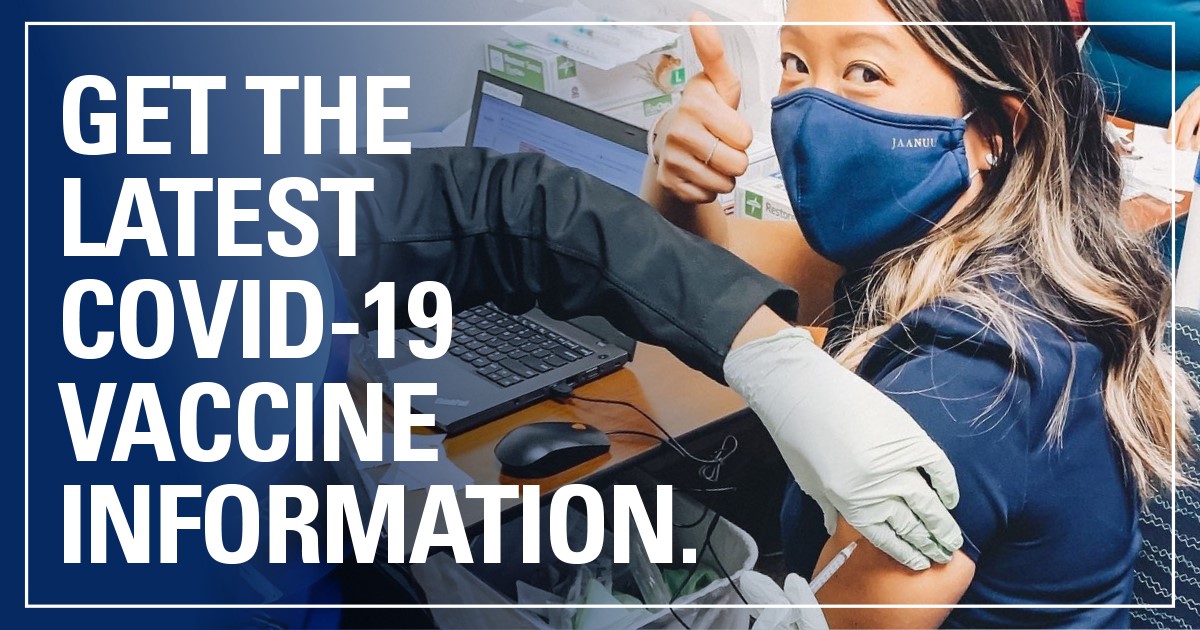A detailed public service announcement photograph shows an Asian woman with dark hair and blonde highlights seated in a chair, receiving a COVID-19 vaccination. She is wearing a blue shirt and a matching blue mask. Her right thumb is up in a gesture of approval while her left arm is being vaccinated. The nurse administering the shot is only partially visible, with white gloves and black long sleeves covering her arms. 

In the foreground, there's a brown table with an open black laptop and a black mouse. Below the table, a white-lined garbage can is noticeably full. In the background, a second woman, identifiable only by her abdomen covered in a blue shirt, is seen standing. 

The photograph is framed by a thin white border, and text in the top left corner reads, "Get the latest COVID-19 vaccine information." The overall composition emphasizes the importance of staying informed and making informed health decisions.